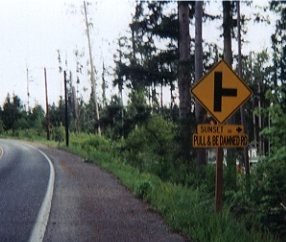This image captures a serene, rural roadway winding through a wooded landscape under a light blue, almost white sky. The photo is taken from the right side of the road, showing just the right lane. The road slightly curves to the left from the bottom left corner of the image, continuing off into the distance with no traffic in sight. A white line delineates the shoulder, which is quite wide and merges into lush, dark green grass and a dirt side that flanks the road.

To the right of the road, there's a yellow diamond traffic sign, indicating a straight road with an intersection ahead on the right. Below this sign, a yellow plaque reads "Sunset Road" with an arrow pointing right, and beneath it, partially blurred, is "Pull and Be Damned Road."

The roadside is bordered by a dense pine forest with a mix of evergreens and other trees, some with leaves still clinging to their branches. The lower vegetation consists of full green bushes and scraggly trees. Telephone poles sporadically line the roadside, further emphasizing the rural, untouched feel of the scene.